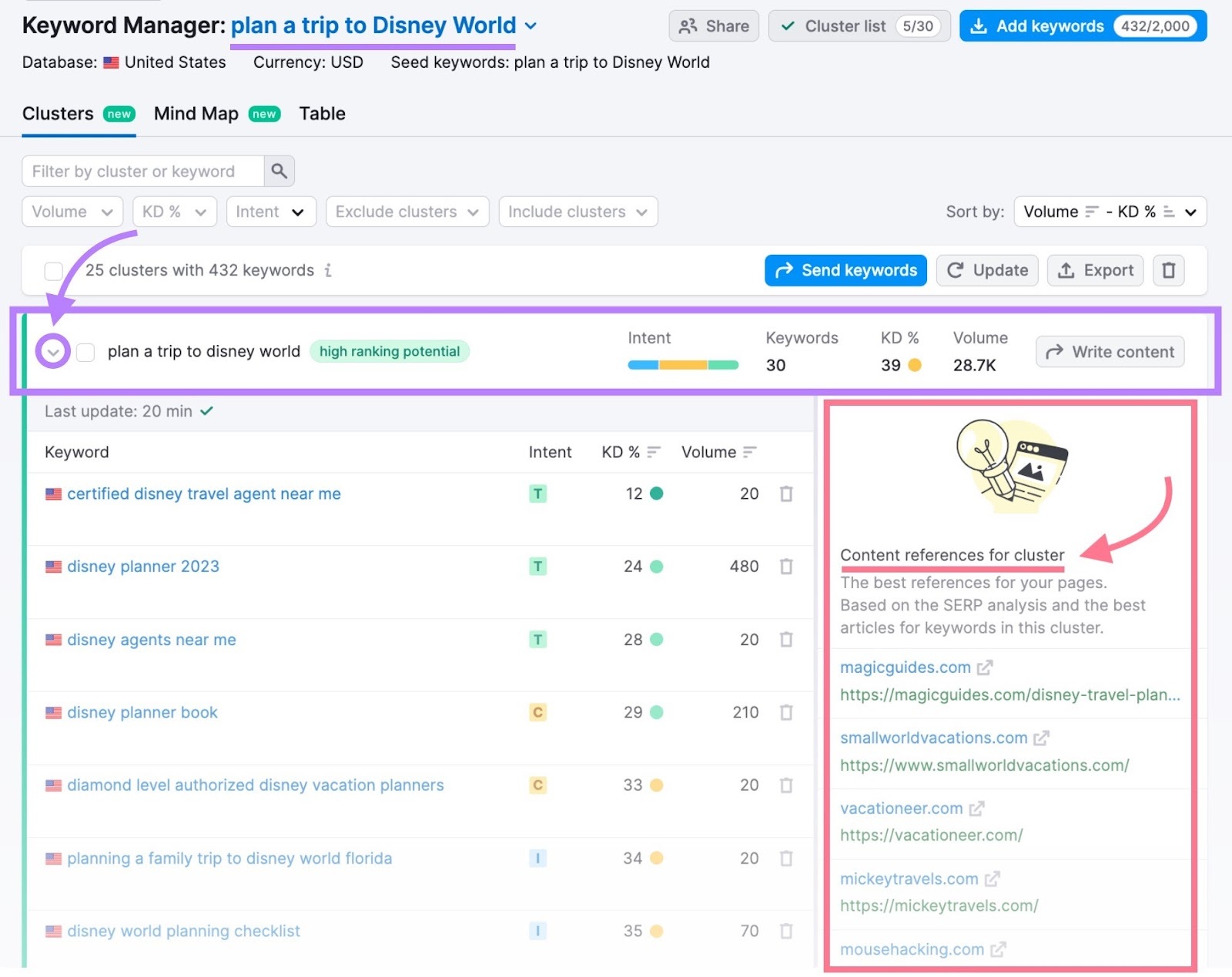Screenshot of a website interface titled "Keyword Manager" featuring a detailed keyword analysis tool. The top left corner reads "Database: United States, Currency: USD" with "Seed Keywords: plan a trip to Disney World." Below this, a green "New" banner highlights the "Clusters" tab, adjacent to other tabs labeled "Mind Map" and "Table." A search bar offers filtering by cluster or keyword.

Highlighted sections include dropdown menus for "Volume," "KD%," and "Intent," along with options to "Exclude Clusters" or "Include Clusters." A prominent purple arrow directs attention to a box outlined in purple that emphasizes "Plan a Trip to Disney World" as having high ranking potential, detailing its intent, keywords, KD%, and volume metrics.